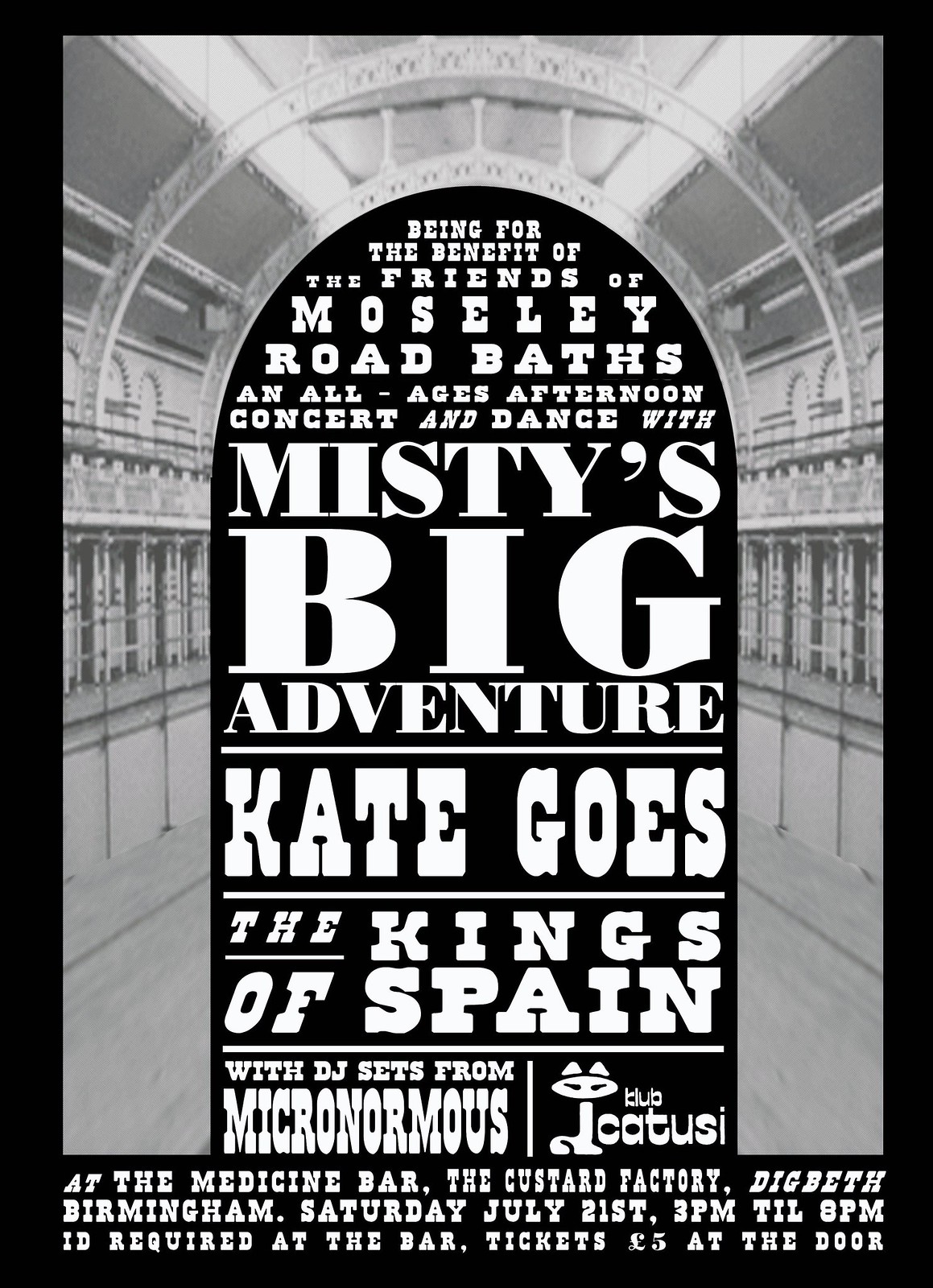This is a detailed poster advertisement for an all-ages afternoon concert and dance event. The poster has a grayscale background featuring a large, intricately designed arched building facade with visible windows and decorative patterns. At the top of the poster, in small white letters on a black background, it reads, "Being for the benefit of the friends of Moseley Road Baths." Below that, it announces "An all ages afternoon concert and dance with Misty's Big Adventure" in large, bold white letters. This is followed by performances from "Kate Goes" and "The Kings of Spain" in slightly smaller white letters. At the bottom, it mentions a DJ set from "Micronormous," and to the right, a caricature of a cat next to the mention of "Club Katusi." The event details at the bottom of the poster state, "The Medicine Bar, The Custard Factory, Digbeth, Birmingham, Saturday, July 21, 3 PM till 8 PM. ID required at the bar, tickets, five pounds at the door."